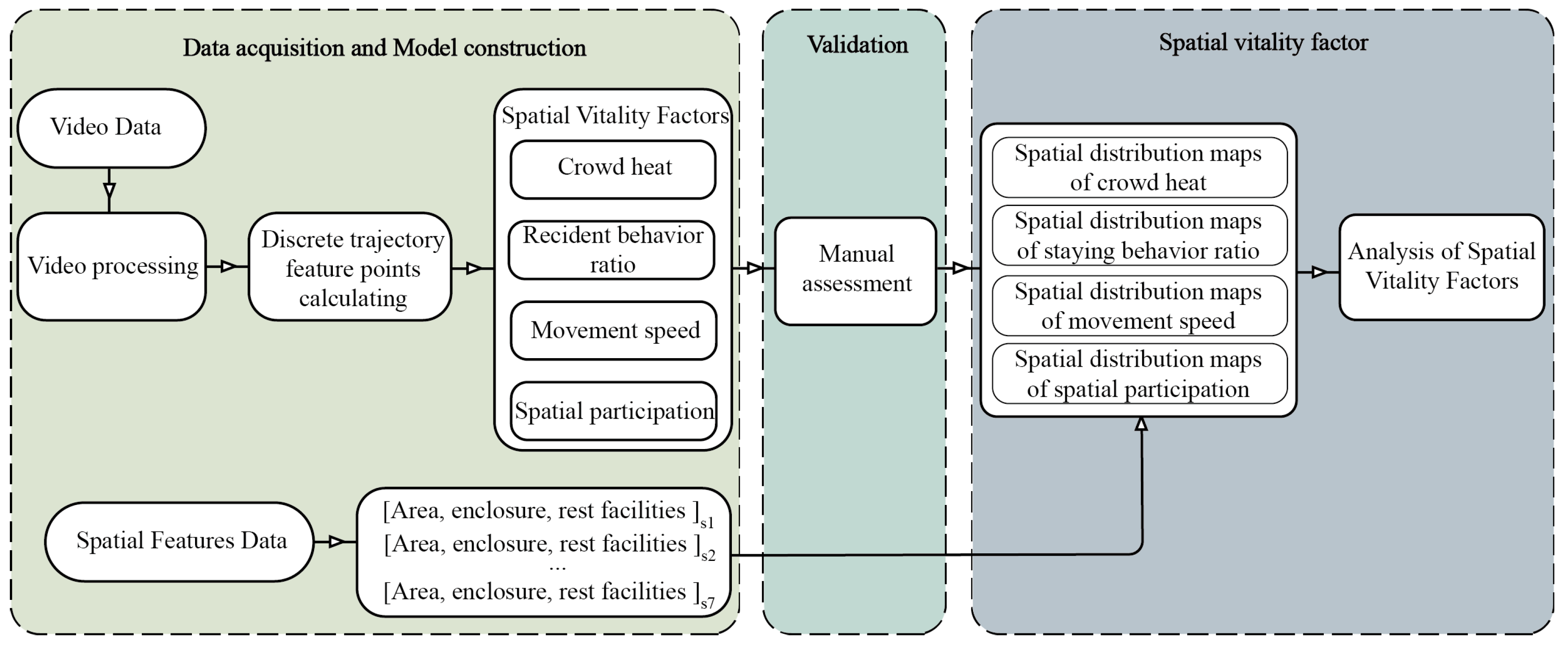The image features an intricately connected series of flowcharts, each housed within a distinct colored rectangular box. On the left, the largest flowchart is set against a green background and titled "Data Acquisition and Model Construction" in black font at the top. This section encompasses a detailed process starting with "Video Data" and progressing through "Video Processing," leading to the calculation of "Discrete Trajectory Feature Points" and incorporating "Spatial Features Data."

This pathway flows into the middle chart, which is narrower and set on a teal background, titled "Validation." Here, the primary focus is on "Manual Assessment," which ensures the integrity and accuracy of the data being processed.

Finally, the rightmost flowchart, larger than the middle but smaller than the first, features a light gray background and is titled "Spatial Vitality Factor." It further elaborates on spatial elements such as "Crowd Heat," "Resident Behavior Ratio," "Movement Speed," and "Spatial Participation." These factors ultimately converge into "Analysis of Spatial Vitality Factors," offering deeper insights into spatial dynamics. The entire flow emphasizes a structured progression from initial data acquisition through rigorous validation to comprehensive spatial analysis.